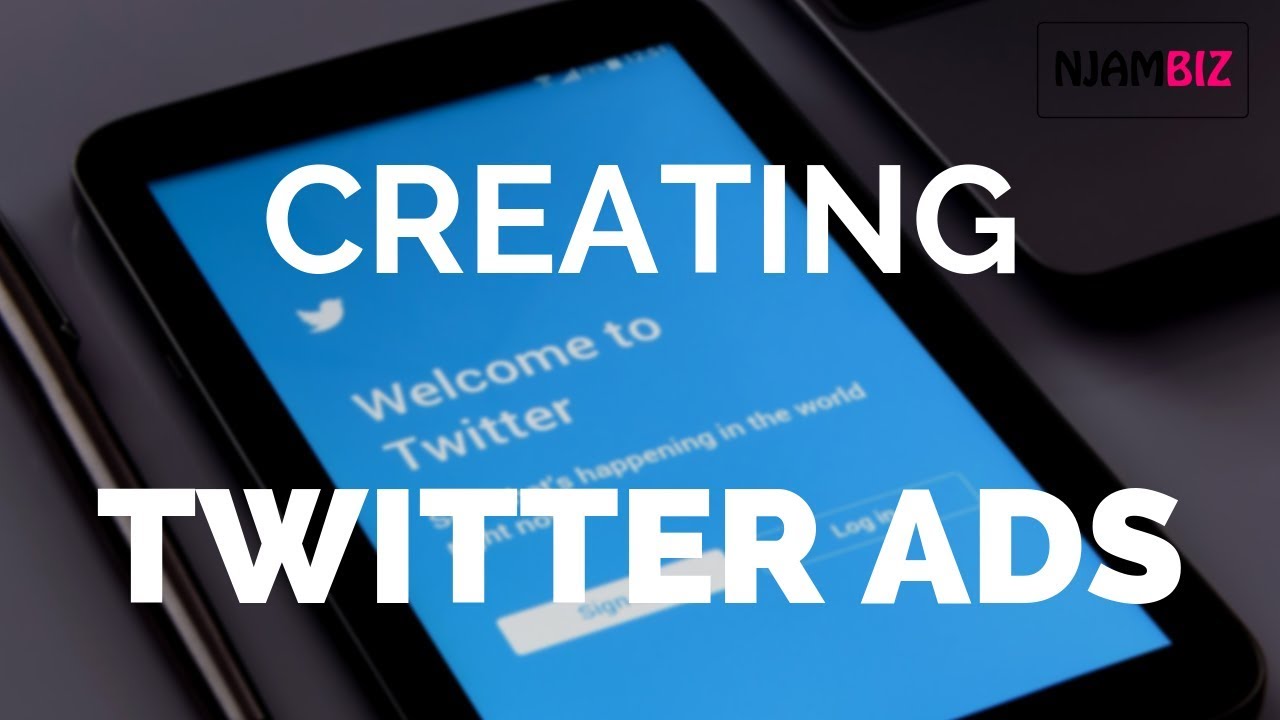This image features an iPad resting on a black surface. Displayed prominently on the iPad's screen, the upper right-hand corner shows the abbreviation "BIZ" in bold, capital red letters. Dominating the center of the screen is the phrase "CREATING TWITTER ADS," written in large, bold, white capital letters. Below this, the words "Welcome to Twitter on the iPad" are visible, albeit partially obscured by the central text. A portion of Twitter's iconic bird logo, set against a blue background, is also discernible. The obscured background text seems to read, "welcome to Twitter. Something's happening in the world," but the exact wording is unclear due to the overlaying text. Additionally, two buttons labeled "Login" and "Sign Up," both in white, are visible on the screen. Behind the capital red "BIZ" text, a partially visible word "N-J-A-M" appears in black, blending into the black surface below and making it difficult to discern fully. This composition suggests a promotional or instructional page related to creating Twitter ads on an iPad.